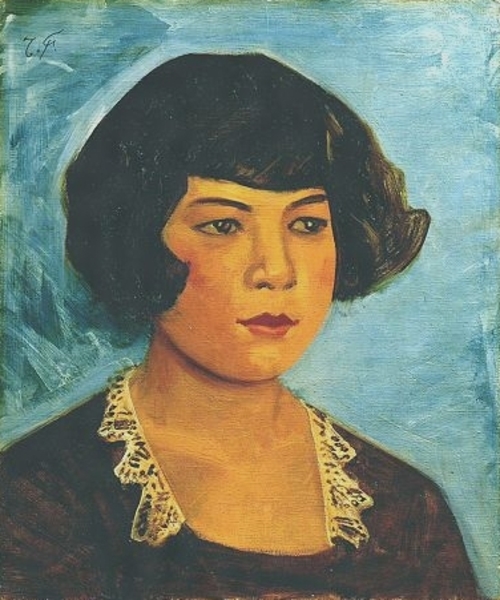This is a vertical, rectangular watercolor painting of a woman in her early to late 20s. The woman appears to be of mixed descent, possibly Asian or Pacific Islander. She has a delicate visage with short, dark brown hair that reaches her jaw and bangs that frame her forehead. Her almond-shaped eyes are dark, and her red lips are pursed, adding a touch of intensity to her expression. Her skin, painted in warm orange and flesh tones, suggests a blend of ethnicities.

She is seated and facing to her left, which is on the right side of the painting. She wears a dark dress with a distinctive white lace collar that extends down in a square shape, ending just above her cleavage. The background is a harmonious blend of various shades of blue, with subtle hints of green, reminiscent of an indoor setting but abstract in its execution.

The painting's texture is noticeable, with visible brush strokes along the edges, enhancing its artistic authenticity. Although there is no explicit text in the image, there appears to be a signature in the top left corner, potentially marked "TF". The primary colors in the composition are the blue hues of the backdrop, the dark tones of her hair and dress, and the orange to yellow shades of her skin.